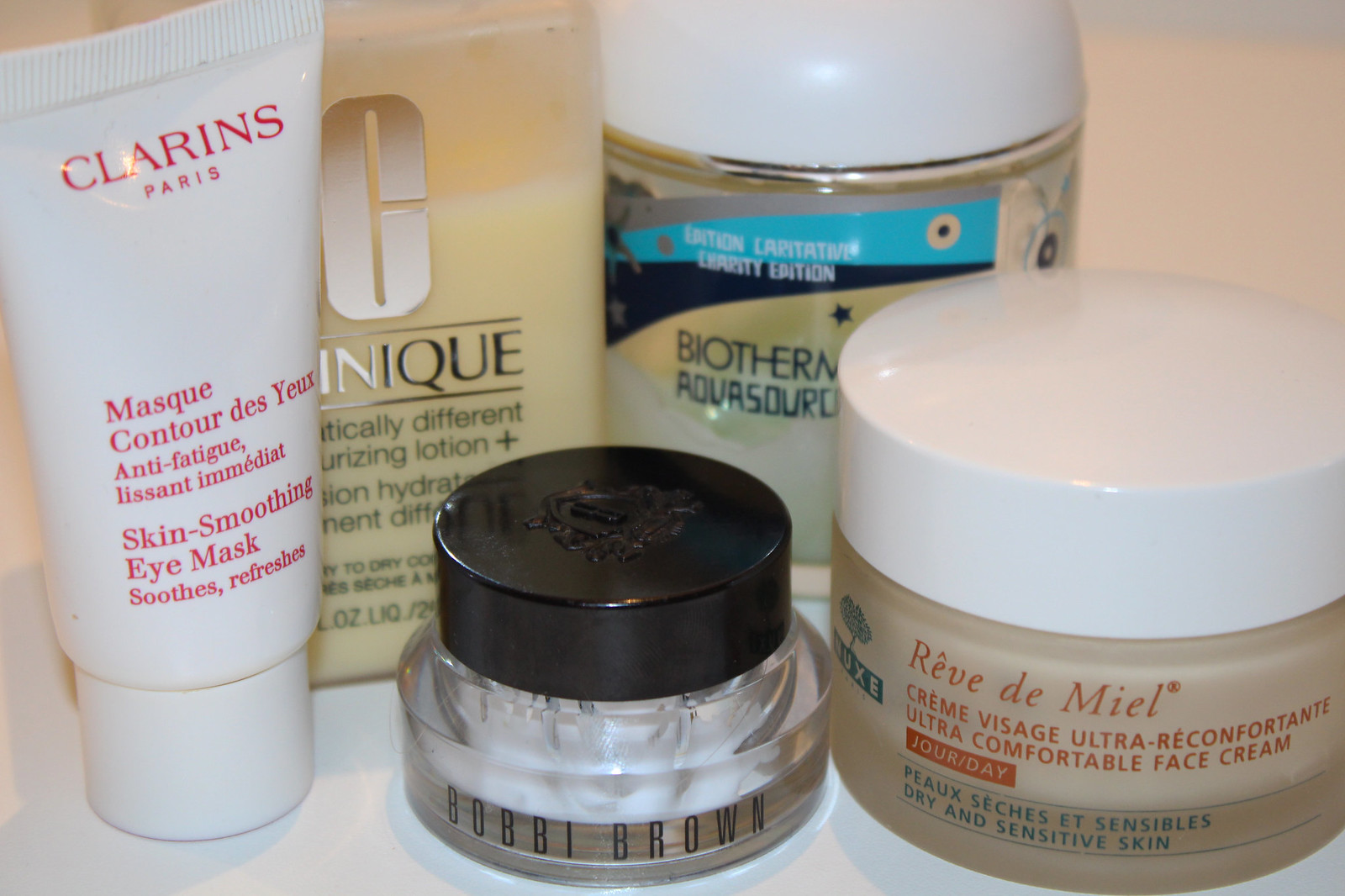The image features a collection of beauty products neatly arranged against a white background. On the far left, there is a white squeeze tube with a cap at the bottom. The red text on the tube reads "Clarins Paris Mass Contour Desio Anti-Fatigue Lassana Mediate Skin Smoothing IMS Soothe Refresh." Adjacent to this tube, partially obscured, is a beige container with the words "Unique" and "moisturizer" visible, and mentions of hydration benefits.

Next in the lineup is a plastic bottle with a round white lid, adorned with a turquoise, black, and tan label that states "Biotherm Aqua Source." Directly in front of this bottle is a glass container featuring a black top, labeled "Bobbi Brown" at the bottom.

To the right, there's a brown jar with a white round lid. The red text on it reads "Reve de Miel Cream Visage Ultra Reconform Nante Ultra Comfortable Face Cream Jourday," with additional blue text indicating it is suitable for "Processed Sensible Dry Skin."

Each product is positioned to highlight its unique packaging and brand identity, creating a visually appealing and informative display of beauty skincare items.